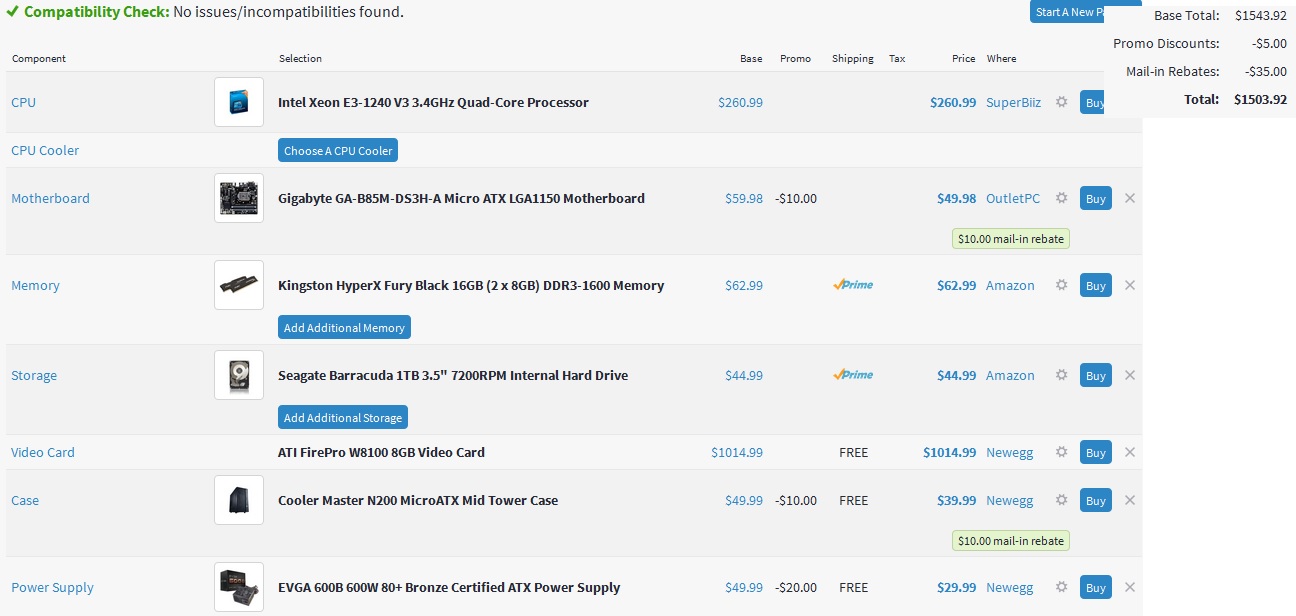This image is a screenshot from a computer hardware assembly website that resembles partpicker.com. The platform allows users to assemble their own computer by selecting individual components, ensuring compatibility, and providing purchasing options. The website features a clean, white and light gray color scheme with black text, supplemented by clickable blue links.

At the top left of the screenshot, a green checkmark followed by green text indicates that a compatibility check has been completed, displaying "No issues/no incompatibilities found." Below this section, a left-hand column lists the various computer components necessary for a build: CPU, CPU cooler, motherboard, memory, storage, video card, case, and power supply.

To the right of this list, there is a "Selection" column where the specific components chosen by the user are displayed, including the selected processor, motherboard, memory sticks, hard drive, etc. Next to this column, there is a "Base" column, presumably indicating the base price of each component.

Subsequent columns provide additional details: "Promos" for any promotional deals, "Shipping" for shipping costs, "Tax" for tax information, and finally, the price at a specific retailer. Each listed component features a blue "Buy" button for easy purchasing.

Overall, this detailed screenshot provides a comprehensive view of the process of selecting and assembling computer components, with a focus on compatibility and cost-efficiency.